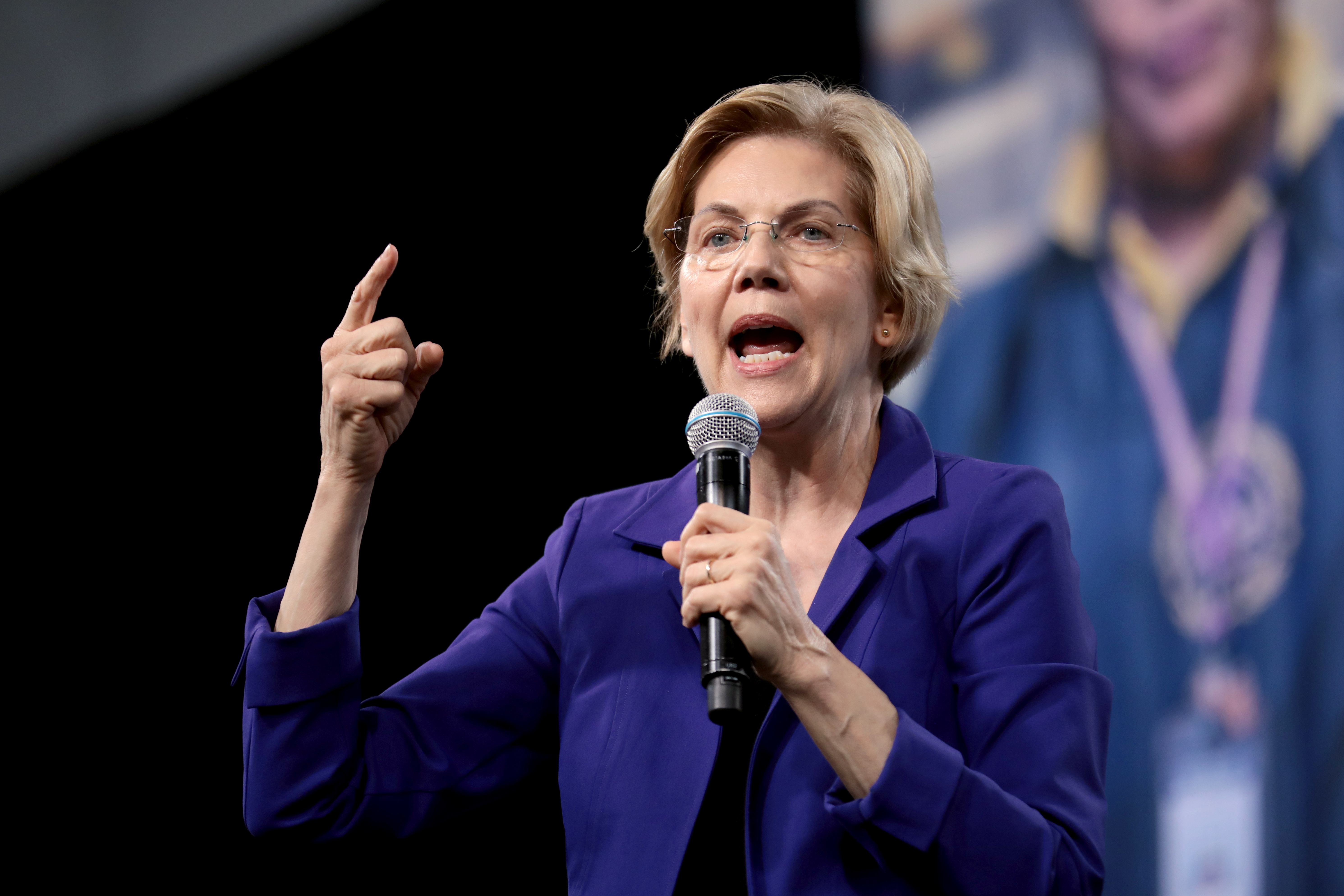This image captures Senator Elizabeth Warren passionately speaking, with her right hand raised, index finger extended as if making a crucial point. In her other hand, she holds a black microphone up to her open mouth, emphasizing her speech. Senator Warren, identifiable by her short blonde hair and thin rectangular glasses, is dressed in a purple suit jacket over a black shirt. She is adorned with stud earrings and a wedding ring on her finger. The backdrop features a large, blurred image, possibly of a graduate, which appears to be superimposed on the scene, while the left side of the background fades into a mostly black expanse with a touch of gray in the upper corner.